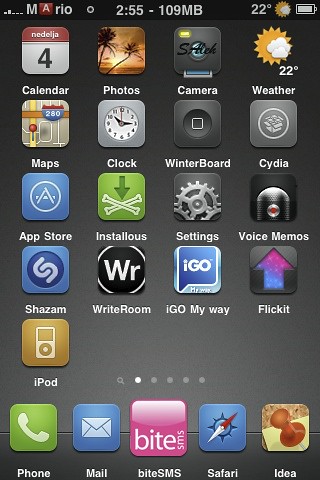The image is a detailed screenshot of an iOS device's home screen. At the top of the screen, there's a black rectangular banner displaying "Mario," followed by "255," and "109 MB," with a fully charged battery icon and the temperature "22 degrees" accompanied by a sun and cloud symbol. The home screen displays various app icons organized in six rows and a bottom dock. Prominent apps include Calendar (showing the date as "4"), Photos (with a palm tree icon), Camera, Weather (showing 22 degrees and a sun with a cloud), Maps (highlighted with route 280), Clock (reading 10:15), Winterboard, Cydia, Apple App Store, Installous, Settings (represented by a cogwheel), Voice Memos, Shazam, Right Room, Igo My Way, Flick It, and iPod. The bottom row, or dock, consists of icons for Phone, Mail, ByteSMS, Safari, and an app labeled 'Idea.' The background features a gradient, transitioning from black at the top to gray at the bottom.